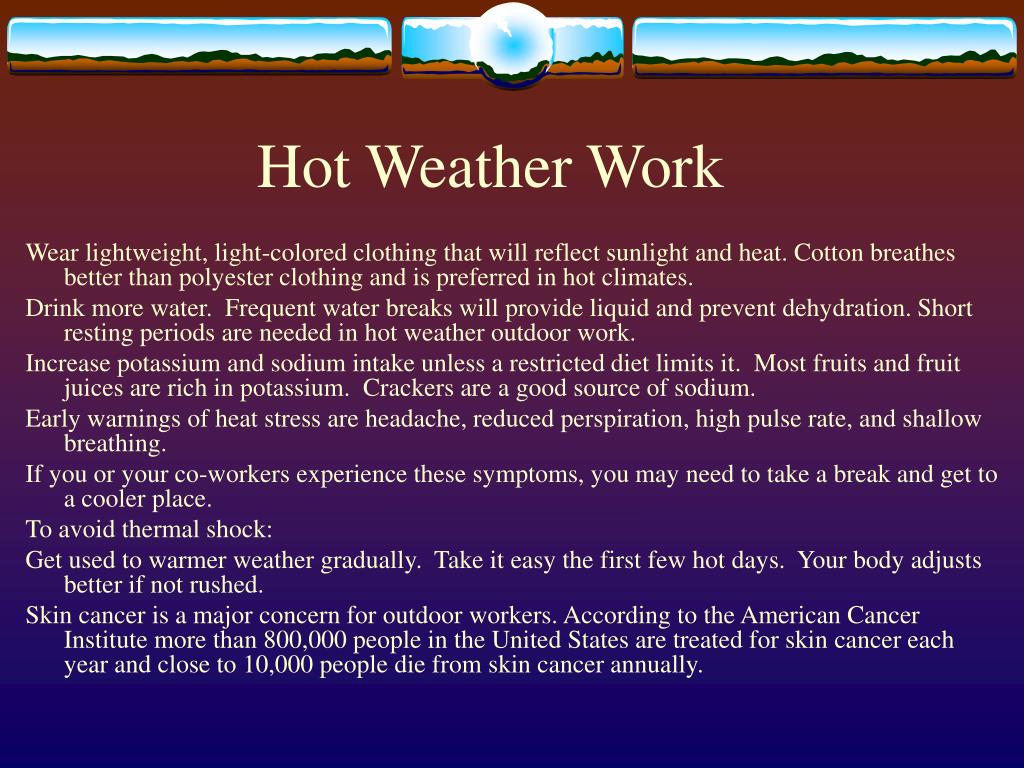The image features a rectangular, PowerPoint-like slide with a background gradient transitioning from maroon at the top, through a pinkish-purple center, to a bluish-purple at the bottom. At the very top, there's a collage of three rectangular images showing a sequence of the sky, a tree line, and a dirt area, with a central circle replicating portions of these images. 

Below this collage, large light-yellow text spells out the title "Hot Weather Work." The main body of the slide contains many lines of detailed white text offering comprehensive advice for working in hot weather. It covers topics such as wearing lightweight, light-colored clothing to reflect sunlight and heat, preferring cotton over polyester for breathability, staying hydrated with frequent water breaks, and taking short resting periods. It also advises to increase potassium and sodium intake, identifies early warnings of heat stress (headache, reduced perspiration, high pulse rate, shallow breathing), and recommends gradually adjusting to warmer weather to avoid thermal shock. The slide emphasizes the importance of skin cancer awareness, noting that over 800,000 people in the U.S. are treated for it annually, with close to 10,000 deaths. The top half of the slide is primarily brown, transitioning to dark blue at the bottom, with the mentioned text prominently displayed across multiple lines.